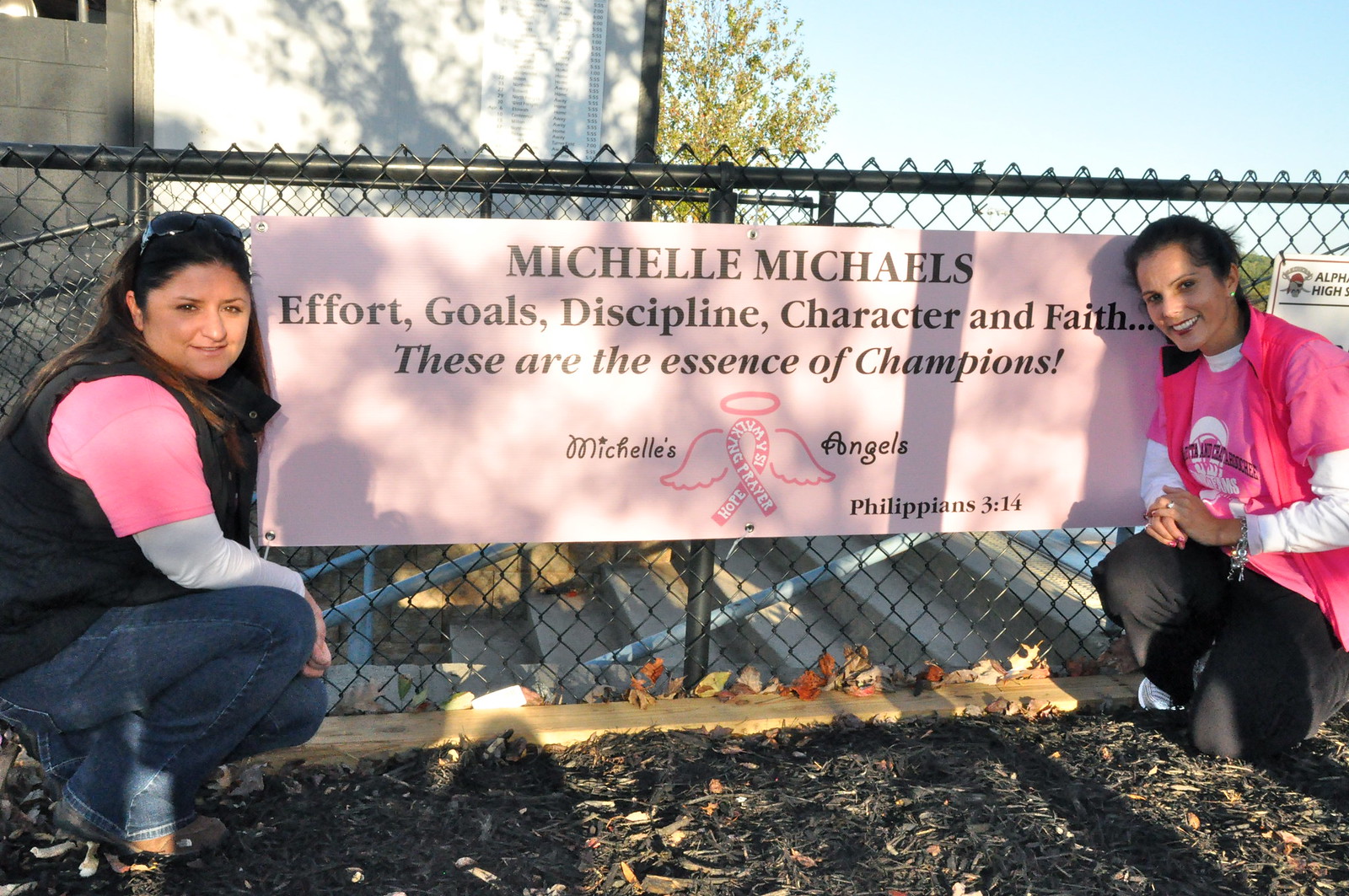In this rectangular photograph, two women are crouched down on dark mulch in front of a black, waist-high chain-link fence, showcasing a pink sign between them. Both women are smiling at the camera and appear to be part of a commemorative event for "Michelle Michaels' Champions." The woman on the left is dressed in blue jeans, brown shoes, a white long-sleeved t-shirt with a short-sleeved pink t-shirt over it, and a black vest. She has shoulder-length brown hair held back by sunglasses. The woman on the right has her slightly darker hair pulled back, is wearing black pants, and has a similar outfit—pink t-shirt over a white long-sleeved t-shirt with a pink or black vest. The sign between them is predominantly pink with black text that reads, "Michelle Michaels. Effort, Goals, Discipline, Character, and Faith. These are the essence of champions." It features a pink ribbon with angel wings and a halo, labeled “Hope is a walking prayer,” and flanked by the words "Michelle's Angels". At the bottom, it cites Philippians 3:14. The fenced backdrop, with a blue sky, a tree, and part of a building, frames this heartfelt tribute.